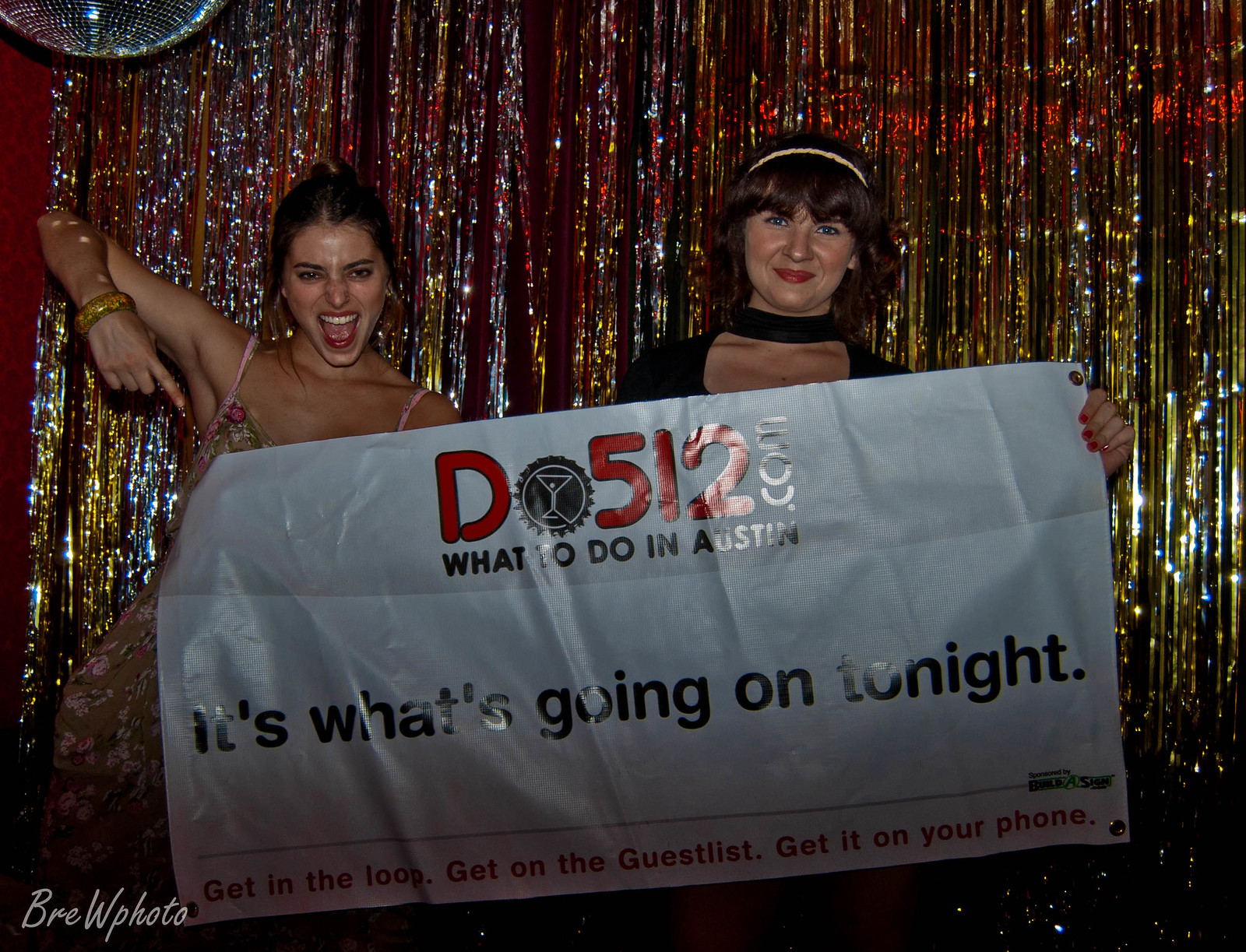In the image, two girls pose together holding a white sign. Behind them, on the top left, a disco ball reflects festive light amidst a backdrop of shiny, plastic streamers that give a party-like atmosphere. The girl on the left is dressed in a short, strapless floral dress, has brown hair, and wears lipstick. The girl on the right dons a black dress and has black hair with makeup. Both are White women. The sign they hold reads: "do512.com - What to do in Austin." Below, it states: "What's going on tonight? Get in the loop, get on guest list, get it on your phone."